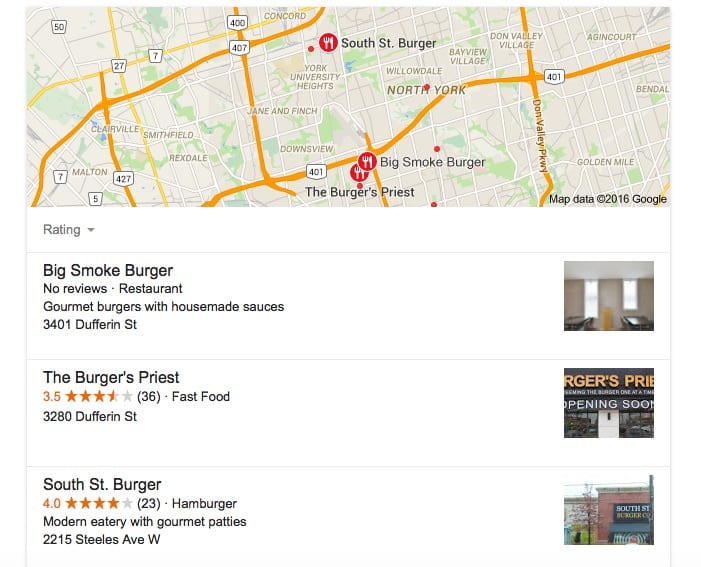This image is a cropped screenshot from a website, focusing on a small section of detailed information. At the top of the screenshot, there's a Google Map displaying a section of America from the year 2016. The map features red circles with white knife and fork icons, marking specific locations.

Beneath the map, there are three highlighted restaurant listings, each accompanied by a brief description and a thumbnail image. All three establishments specialize in burgers:

1. **Big Smoke Burger**: Known for Cormier Burgers with house-made sauces. The thumbnail depicts the interior of the restaurant, suggesting a cozy dining atmosphere.
2. **The Burger’s Priest**: This is a fast-food restaurant with a 3.5-star rating out of 5. The thumbnail shows the front of the shop, indicating its location and exterior appearance.
3. **South Street Burger**: A modern eatery offering gourmet patties with a 4-star rating out of 5. The accompanying thumbnail image is a street view of the restaurant's exterior.

This screenshot captures a focused and informative snippet about these burger restaurants, providing essential details and visual cues for each location.